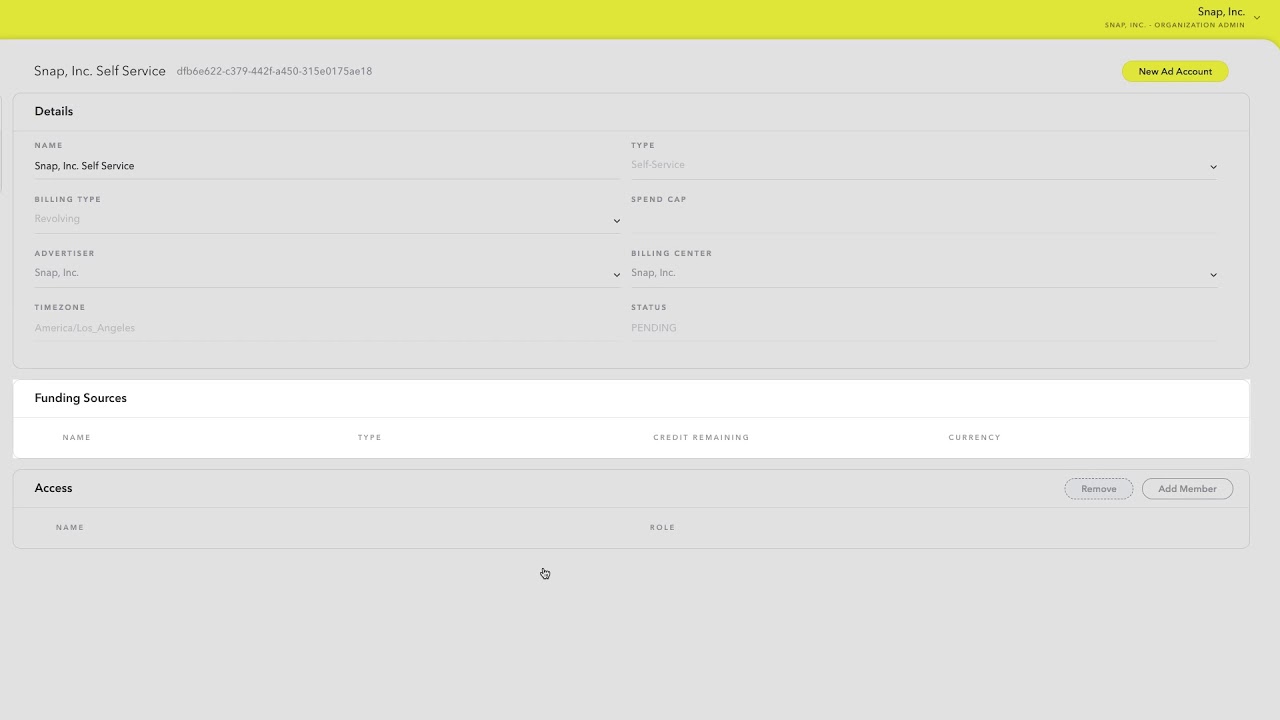This is a detailed caption for the screenshot of the website dashboard:

"Screenshot of the Snap Inc organizational dashboard. At the top, a yellow bar spans across the screen. The top-right corner displays 'Snap Inc,' accompanied by 'Snap Inc Organizational Admin' below it, with an adjacent drop-down menu. Just below the yellow bar, there is a heading 'Snap Inc Self-Service' along with an associated code. Below this heading, the dashboard is divided into three sections: 'Details,' 'Funding Sources,' and 'Access.'

In the 'Details' section, there are four listed items. The first item reaffirms 'Snap Inc Self-Service,' followed by another labeled as 'Type,' which specifies 'Self-Service.' The sections titled 'Funding Sources' and 'Access' contain empty fields beneath their headers, indicating areas that await further information."